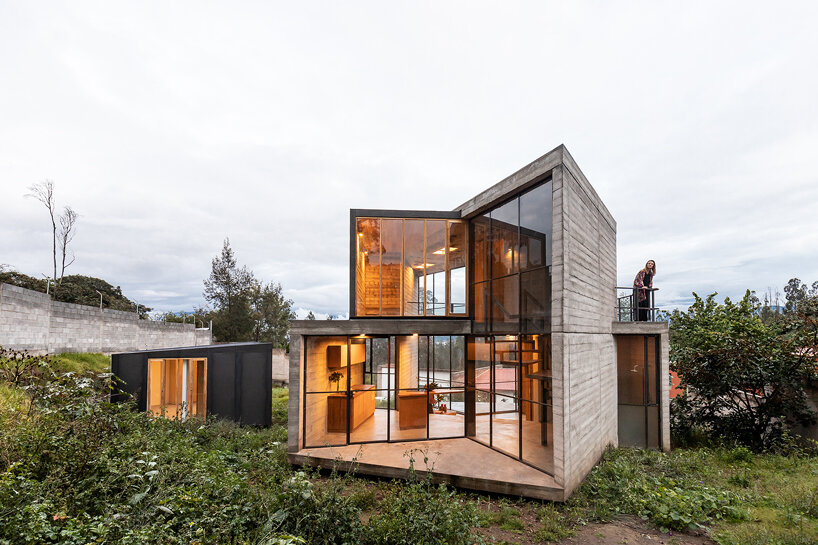In this image, we see an extremely modern and unique house situated in a remote, rural area with no other homes in sight. The house is architecturally distinct, composed of four cube-like structures made primarily of glass, allowing a full view of its wood-toned, yellow and brown interior. The house has two stories, with visible rooms including a kitchen and an upstairs bedroom. Large, glass doors and windows dominate the structure, though there are two solid gray brick walls and a concrete foundation. To the left of the house, there is a small, black shed-like room amidst scattered bushes and trees. The picturesque landscape, heightened by a clear blue sky filled with white clouds, suggests a high-altitude location, possibly on a mountaintop with an expansive, unseen view below. On the right side of the house, a woman stands on the balcony, hands on the rail, gazing into the distance, adding a sense of life to this luxury home that resembles something one might find listed on Airbnb.